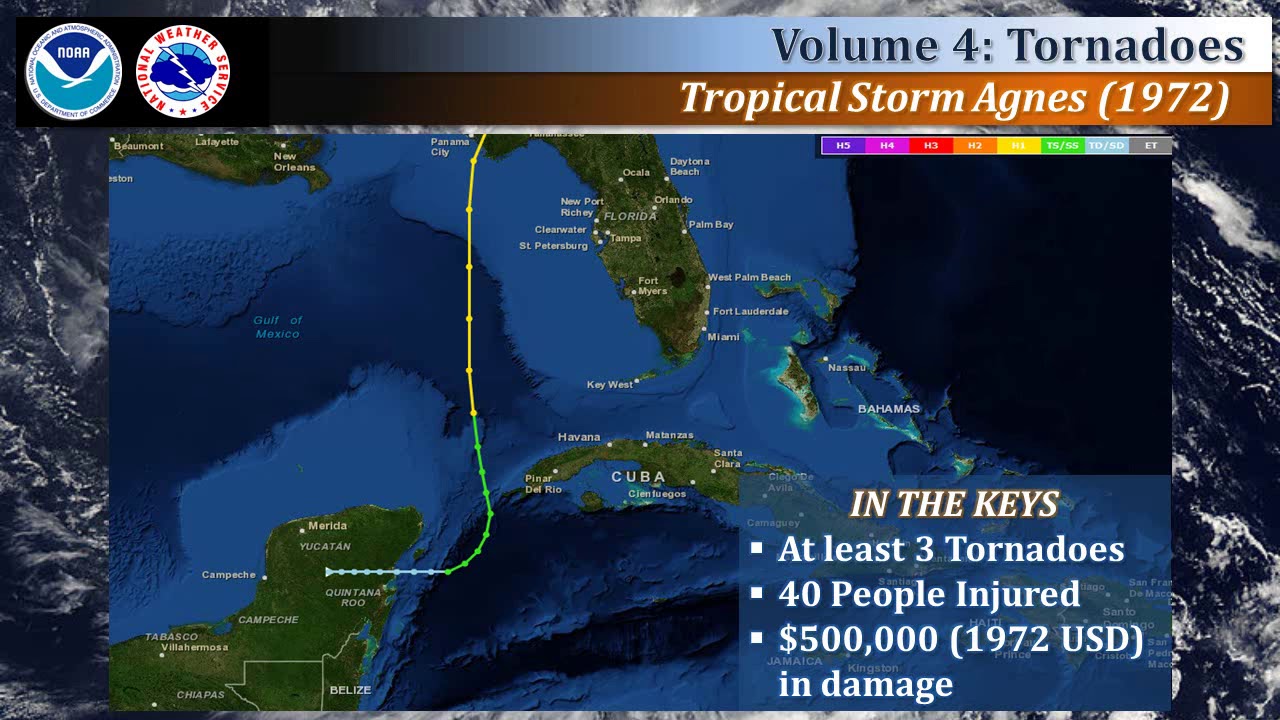The image is a screen capture of a webpage, showing a detailed weather map that includes regions of the United States, Cuba, and the Gulf of Mexico. Centered prominently is Cuba, with the Florida peninsula extending from the top middle, covering about one-third of the state. Positioned on the bottom left are scattered islands, and spanning across the map are multiple shades of blue representing the ocean. A yellow and green trajectory line marks the path of Tropical Storm Agnes, which traveled from the Yucatan Peninsula up to Panama City, Florida.

At the top left corner, there are two circular icons: the first displays the National Weather Service logo in white and blue, and the second features the NOAA logo in similar colors. A blue and brown banner across the top reads "Volume 4, Tornadoes" in black text, followed by "Tropical Storm Agnes (1972)" in white text. In the bottom right corner, a pop-up rectangle provides specific event data: "In the Keys, at least three tornadoes, 40 people injured, $500,000 in damage (1972 U.S. dollars)." The entire image measures approximately 8 inches wide by 5 inches tall.